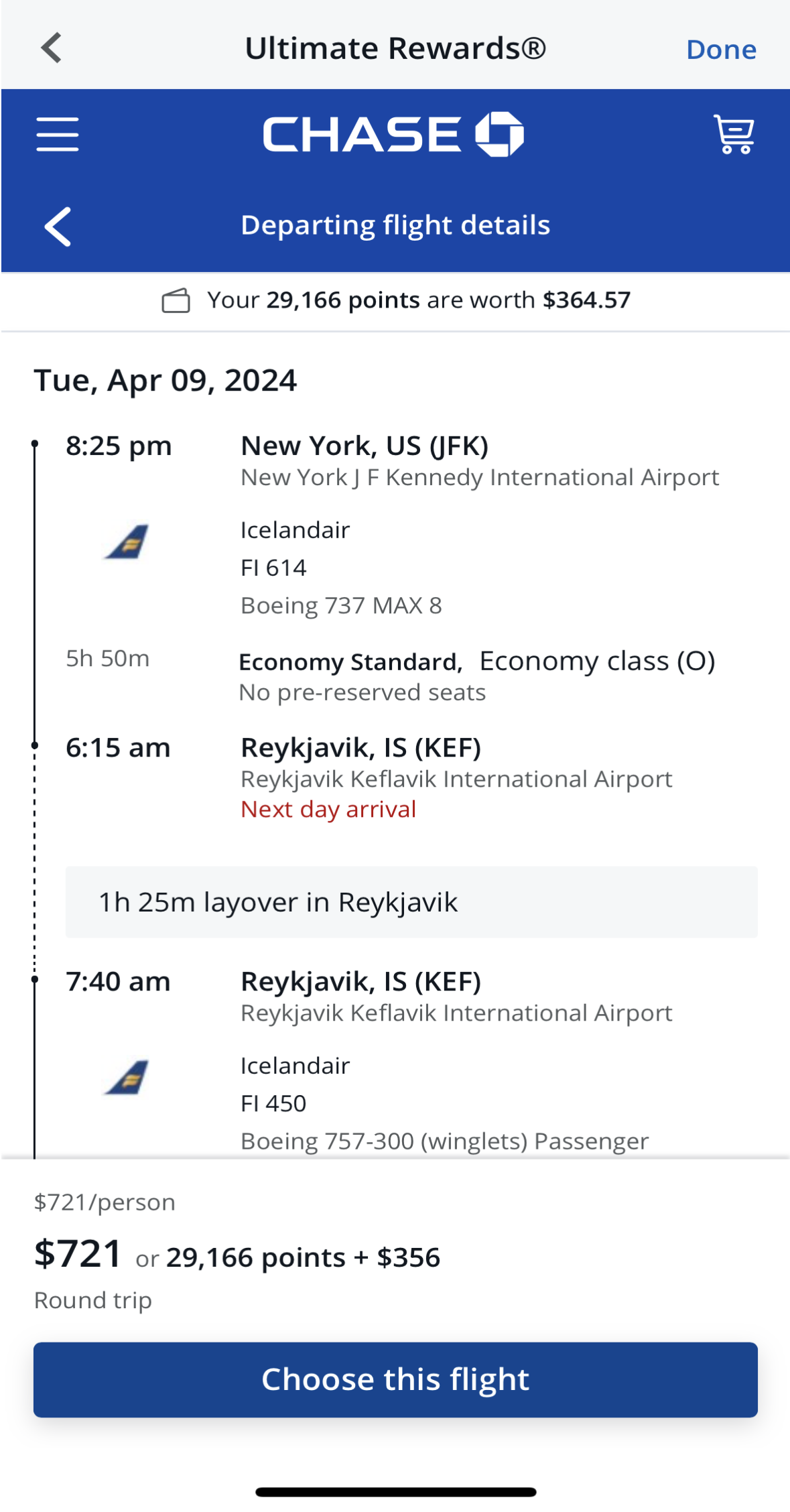This screenshot displays a Chase Bank page with various details related to a departing flight. 

At the top, there is a blue navigation bar featuring the white Chase Octagon logo in the center. On the left side of the bar, there is a menu button represented by three horizontal lines, while the right side features a cart icon.

Below the navigation bar, the page header reads "Departing Flight Deals." To the left of this header, a back arrow is visible, presumably for navigation purposes.

Directly below the header, the page displays the user's points balance, stating, "Your 29,166 points are worth $364.57."

Moving further down, the date "Tuesday, April 9, 2024" is listed, followed by a section titled "Flight Information."

The flight information indicates the following details:
- Departure Time: 8:25 PM
- Departure Location: New York, US, JFK
- Airport: John F. Kennedy International Airport (JFK)
- Airline: Iceland Air
- Flight Number: FL614
- Aircraft: Boeing 737 MAX 8

At the very bottom of the page, there is a blue button with white text that reads "Choose This Flight," providing an option for the user to select this particular flight.